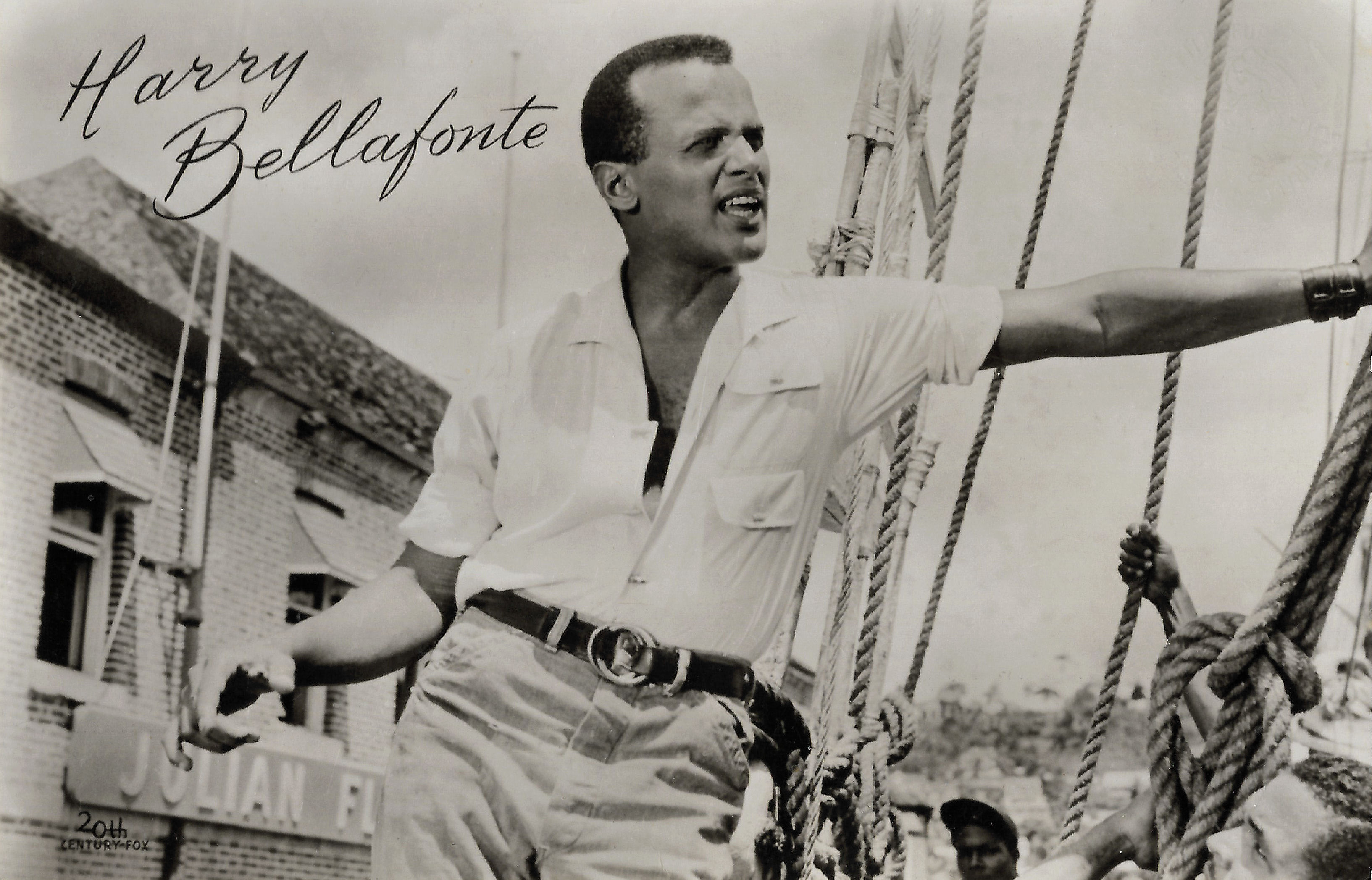This black and white photograph captures a young Harry Belafonte, likely on an album cover, leaning confidently against thick ship ropes on a boat. His short, curly hair is neatly styled, and he gazes off into the distance rather than directly at the camera, exuding a sense of contemplation. Harry is clad in a partially unbuttoned white shirt with sleeves rolled up to his biceps, and jeans secured with a black belt. The composition reveals additional figures and maritime details such as tied knots and ropes extending upwards, enhancing the nautical theme. Notably, the top left corner of the image features his name, "Harry Belafonte" in black script, while the bottom left corner displays the text "20th Century Fox". This evocative scene captures Belafonte in a moment of calm and introspection, possibly referencing his famous songs like "Deo".